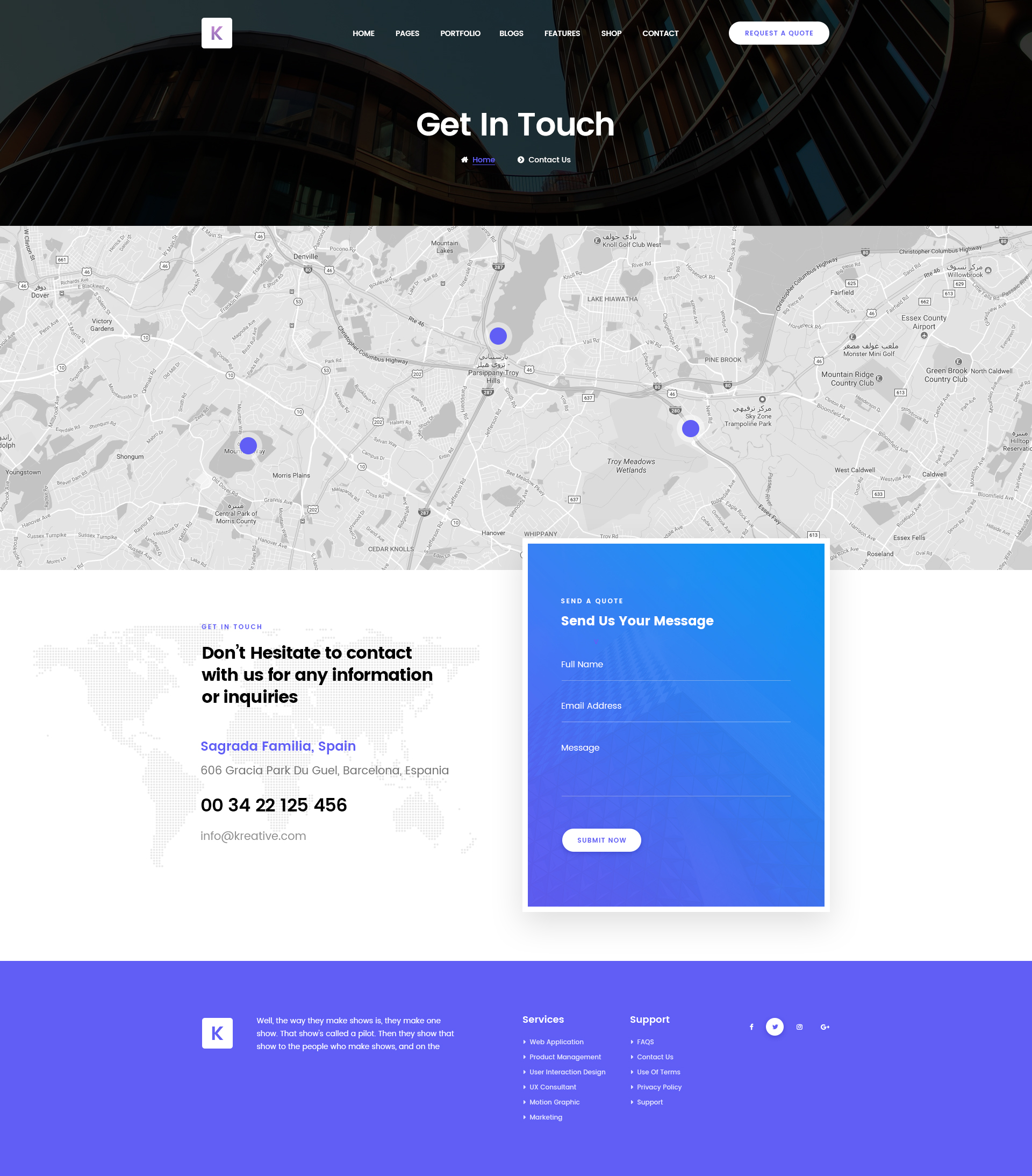The image features a detailed and dynamic webpage layout with a Roman Colosseum-themed header. The top two inches of the image are dominated by a visually striking, darkened depiction that resembles the Roman Colosseum, particularly pronounced on the right side and somewhat on the left. Overlaying this background, heading towards the top left, there's a white circle enclosing a gray "K". Approximately an inch to the right, in small white letters, are navigation links that read: Home, Pages, Portfolio, Blogs, Features, Shop, and Contact. Adjacent to these links, a prominent white tab with black and gray text reads, "Request a Quote". 

Beneath these navigation elements, about an inch down, bolded text reads "Get in Touch". Beside this, a blue Home icon accompanies the text "Home" in blue, followed by a drop-down tab titled "Contact Us" in white. Below this section is a detailed map, approximately two inches high, shaded in light gray with darker gray representing water bodies. The map features three blue location pins.

Towards the bottom right, a dark blue square holds the text "Send a Quote" in white on the left side, with "Send Us Your Message" bolded underneath. Below, in smaller white lettering with underlines, are fields labeled "Full Name", "Email Address", and "Message", accompanied by a white tab reading "Submit Now" in gray.

To the immediate left of this form is a section titled "Get in Touch", followed by bolded black text that encourages visitors not to hesitate in contacting the company for inquiries. This section includes detailed contact information.

The bottom of the image is bordered by a two-inch strip in a purplish-blue hue, providing additional details about the company's services and support. This border also includes icons for social media platforms such as Twitter and Facebook, along with other icons. On the left side of this border, there is further information about the company.